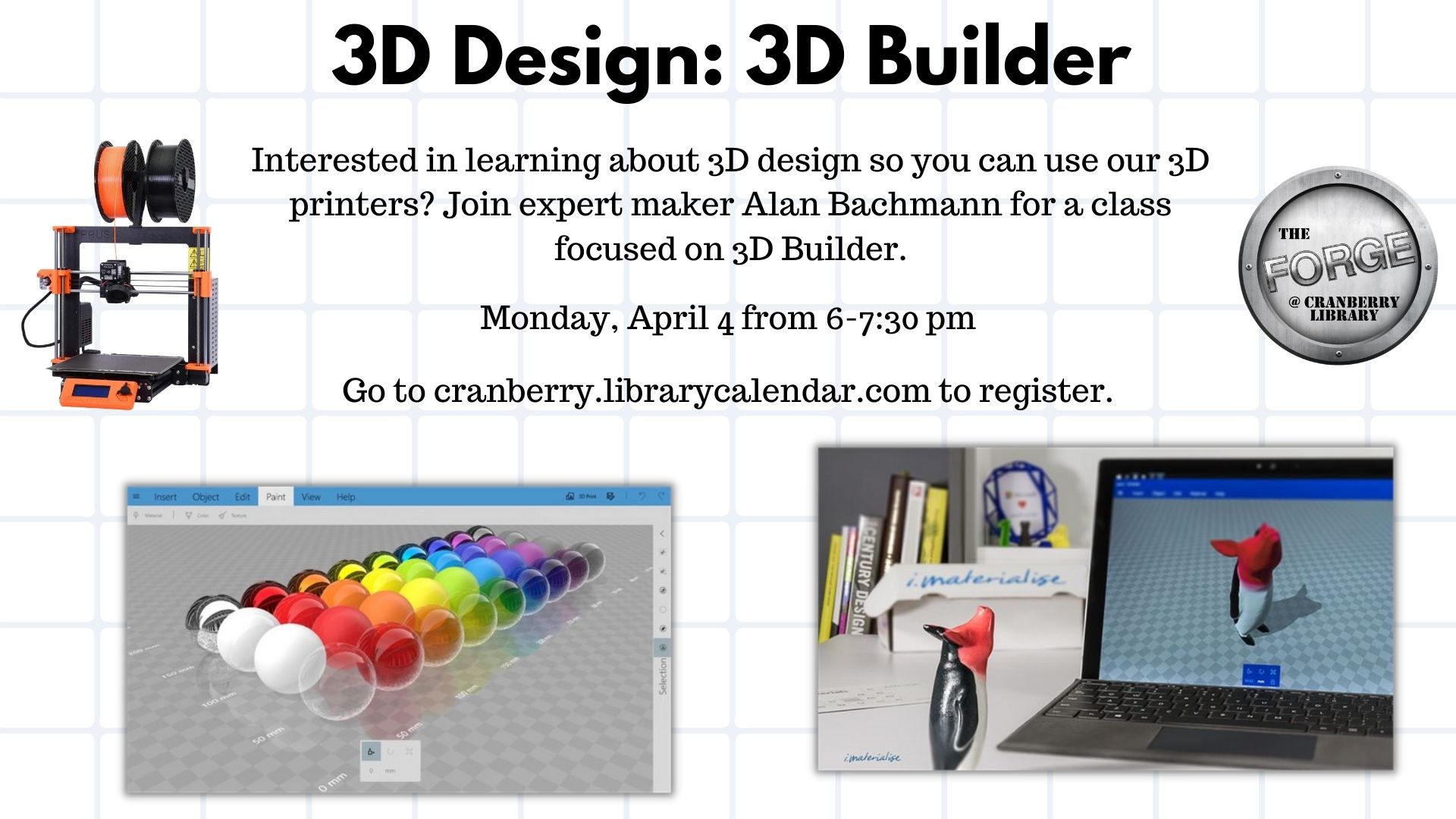The image comprises a promotional flyer for a 3D design class at Cranberry Library. Its design features a modern, minimalist aesthetic, set against a white background adorned with horizontal and vertical gray stripes, creating a grid of small white squares.

At the top of the flyer, bold black text reads: "3D Design, 3D Builder." Just below, an inviting message in the center urges readers: "Interested in Learning About 3D Design? Utilize our 3D printers and join expert maker, Alan Bachman, for a class focused on 3D Builder. Monday, April 4, from 6 to 7:30 PM. Register at cranberry.librarycalendar.com."

The left side of the flyer showcases a stock photo of a 3D printer, predominantly black and orange, highlighting the device's structure. Complementing this is a large gray circle on the right-hand side containing the text "The Forge at Cranberry Library."

The bottom section features two generic stock photos: one on the left displays a collection of variously colored 3D-rendered spheres, reminiscent of early 3D graphics. To the right, another retro-style 3D rendering depicts a laptop with a rendering of a playful penguin on its screen. Accompanying this are a few books positioned on the left-hand side.